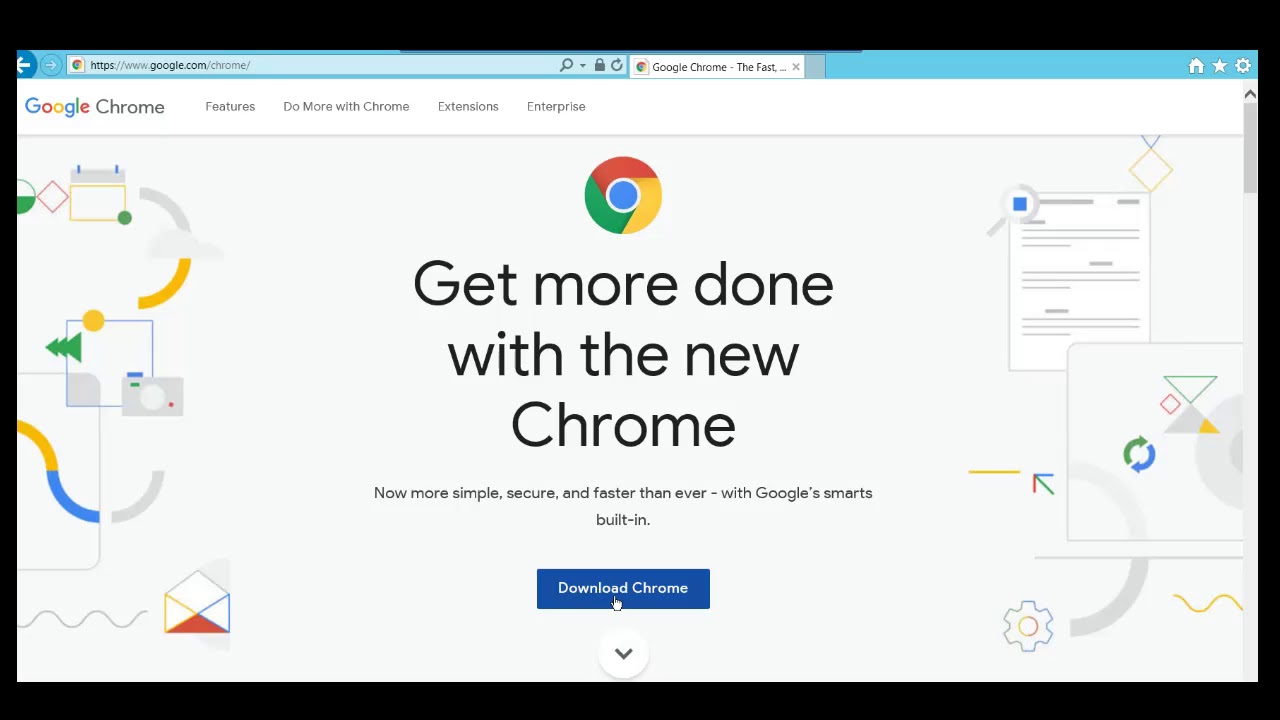The image showcases an older version of the Internet Explorer web browser displaying the Google Chrome download page. The browser's header is characterized by a light blue background, indicating its vintage interface. The URL in the address bar reads "www.google.com/chrome," leading to the Google Chrome landing page.

Prominently featured at the top of the page is the colorful Google Chrome logo, followed by the headline: "Get more done with the new Chrome." Below the headline, the text reads, "Now more simple, secure, and faster than ever with Google smarts built in." Further down, there is a noticeable button with a blue background and white text that says "Download Chrome," inviting users to download the browser.

The background of the webpage is mostly white, contrasting with the black overall background of the image. An arrow icon at the bottom of the screen suggests further navigation or additional information available upon scrolling down.

Transcribed by https://otter.ai